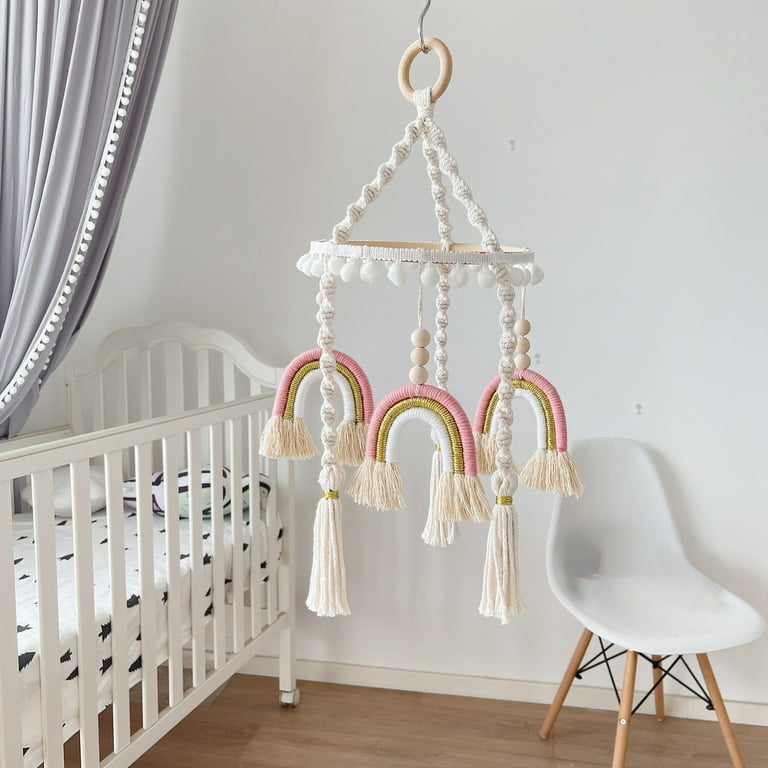This bright, clear photograph captures a beautifully decorated baby's nursery. Dominated by a serene white theme, the room features a white wooden crib placed in the left-hand corner, adorned with sheets that depict tiny black trees and an assortment of pillows, including a black and white striped one and a plain white one. The walls are painted a crisp white, while the floor showcases light-colored natural hardwood. 

A striking detail in the nursery is the intricately hand-crocheted mobile hanging prominently in the foreground. This mobile boasts three rainbows made of pink and gold yarn, interspersed with elegant white twisted crochet elements and small wooden knobs, all suspended from a wood loop. Adding a touch of modernity, a white plastic chair with wooden and steel legs is positioned in the room. Completing the cozy ambiance is a beautiful gray curtain trimmed with decorative ball-like circles, enhancing the nursery's charming and serene aesthetic.